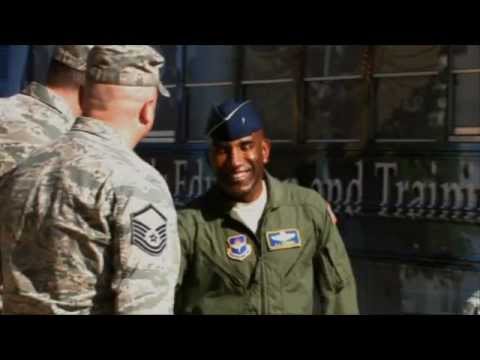This image is a detailed photograph or still shot from a video capturing a group of military personnel in an interaction scene. At the center, a man of black complexion, wearing an olive green flight suit and a navy cap, stands facing the camera with a welcoming smile. His uniform, featuring patches on both sides of his chest and a white t-shirt underneath, indicates his Air Force affiliation. Flanking him on the left with their backs to the camera are two men in camouflaged Army uniforms, distinguishable by their sand and green-patterned attire and military caps. One visibly sports chevrons on his right sleeve. These men of white complexion appear engaged in conversation with the Air Force officer. Behind them looms a structure, possibly a green or gray school bus, prominently displaying partially obscured white text that reads "AND TRAIN." The image is framed by black borders at the top and bottom, adding a cinematic quality to the scene.